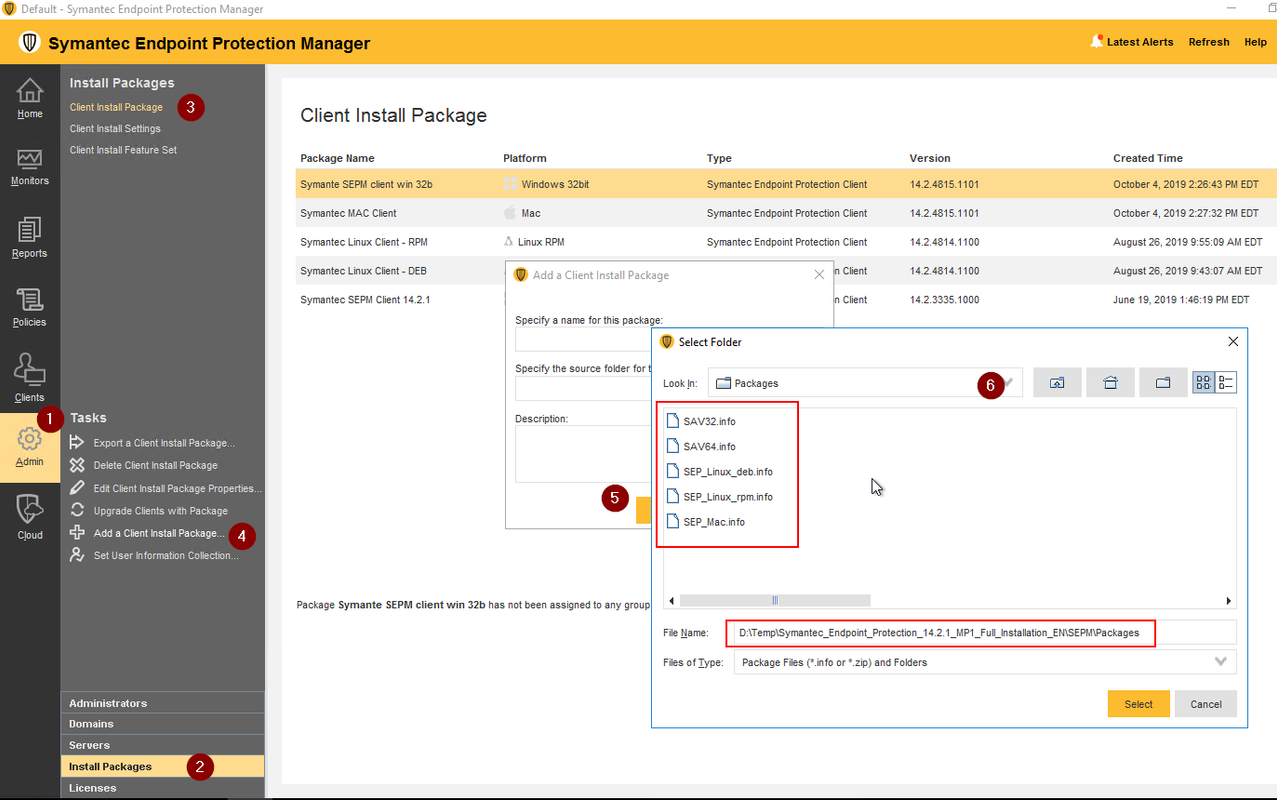This tutorial screenshot showcases the Semantic Endpoint Protection Manager interface, with several key areas highlighted for instructions. 

1. On the left-hand pane, "Admin" is highlighted with a red dot labeled '1'.
2. Further down, '2' marks the "Installed Packages" section.
3. Moving back up, '3' is barely legible, indicating something within the "Client Installed Packages" folder.
4. Highlighted as '4' is an option to "Add a Client Installation Package."
5. The '5' label appears on a pop-up overlay but is obscured by the '6' label, which indicates the need to "Select a Folder."
6. A red square surrounds a list of five files, which are the selectable folders. The specific file needing installation is ringed in red, indicating the required package.